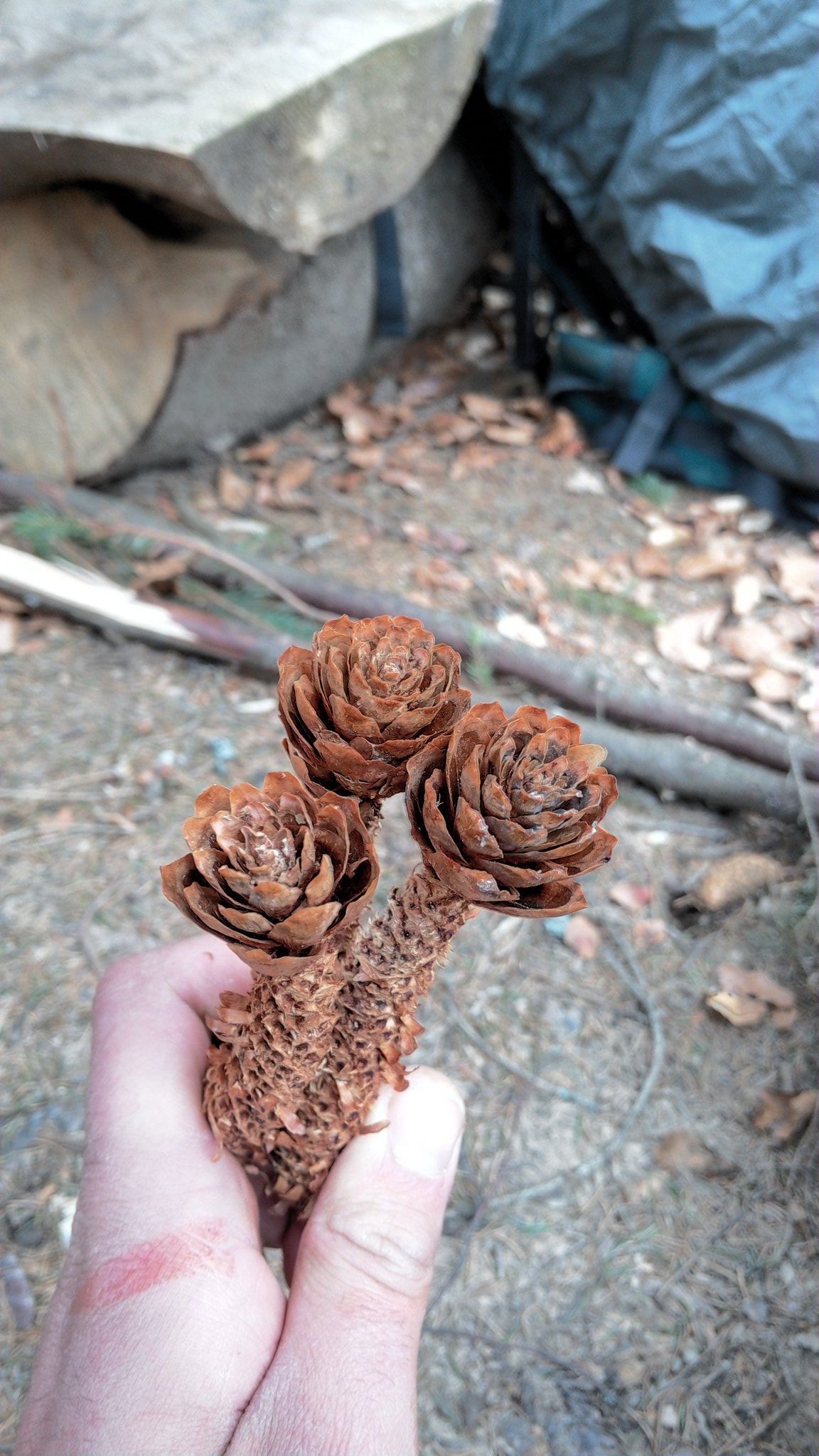This outdoor scene captures the left hand of a fair-complexioned individual prominently holding a twig adorned with three small, brown pine cones that are artfully pulled apart to resemble roses. The image is set amid a ground covered with brown leaves and dirt, indicative of a woodland area. Scattered on the ground are two sticks, a pair of cut logs, and a few smaller branches. In the upper corners of the photograph, a dark blue nylon bag, resembling a tarp or camping gear, is partially visible. The presence of these items, along with the marked logs, suggests that the area might be used for camping or outdoor activities. The individual’s hand showcases a red mark on one of their fingers, adding a touch of personal detail to the scene, which combines elements of nature and human creativity in a rustic setting.